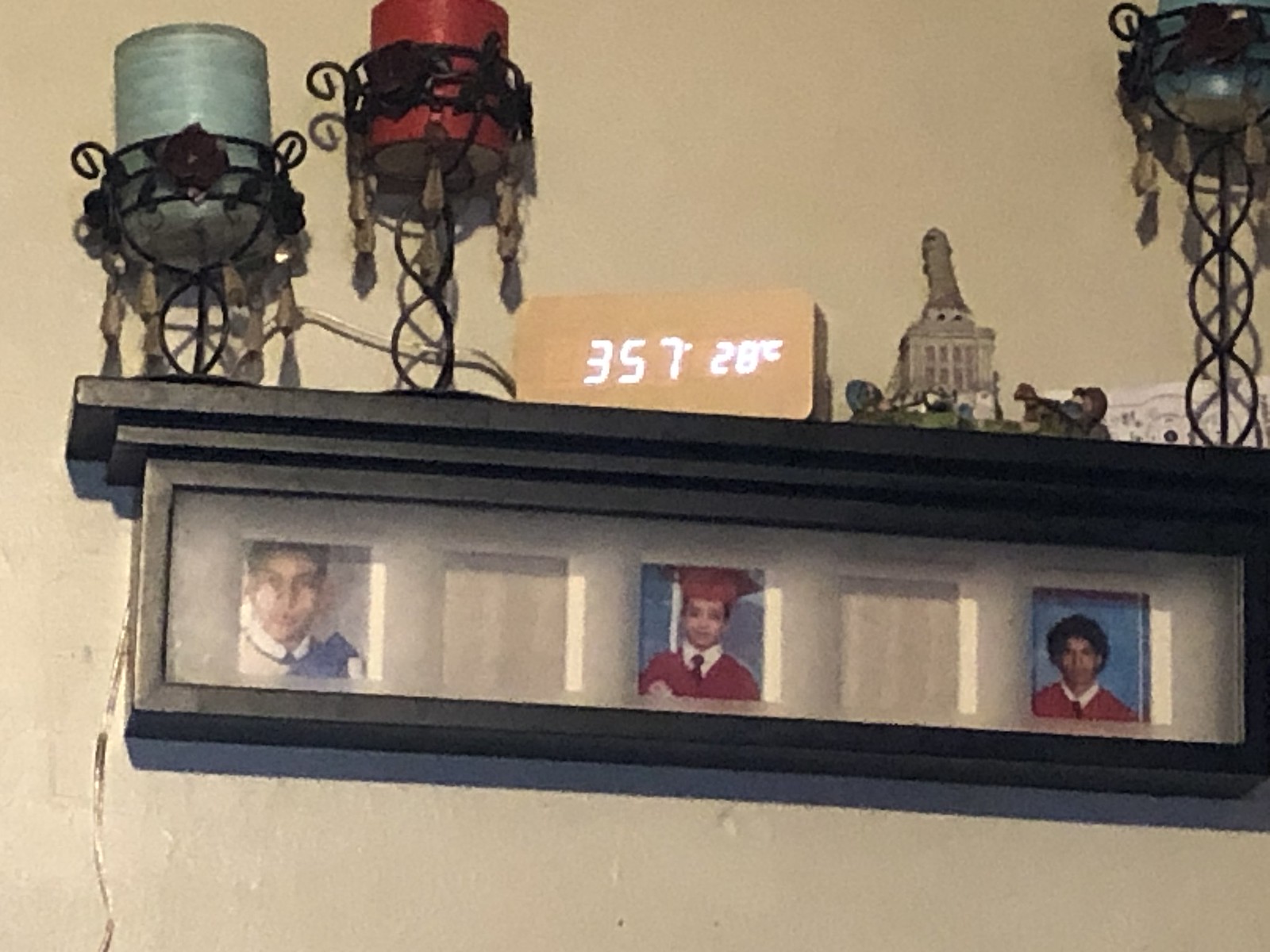A meticulously decorated display mantel is mounted against a slightly textured, off-white, light gray wall. The photo captures the mantel from a slightly upward angle. At the top of the mantel sits a temperature indicator displaying 35.7°C (28°C outside). Elegantly crafted candle holders, resembling circular lampshades, adorn the mantel. The leftmost candle holder, which is greenish-gray, stands next to a slightly taller one with a red candle. The tallest of the set occupies the right side. These candle holders appear to be made from thin, wrought iron, featuring delicate leafy decorations and intricate frameworks at their bases.

The mantel also hosts a collection of small decorative items, including a miniature building and various animal figurines, artfully arranged. Below the mantel, a backlit display showcases images of graduates, most likely relatives of the homeowner. The display comprises five openings, three of which are occupied by photos of graduates in caps and gowns, capturing them from the chest up. A cord hangs down the left side of the wall, adding an additional rustic touch to the scene.